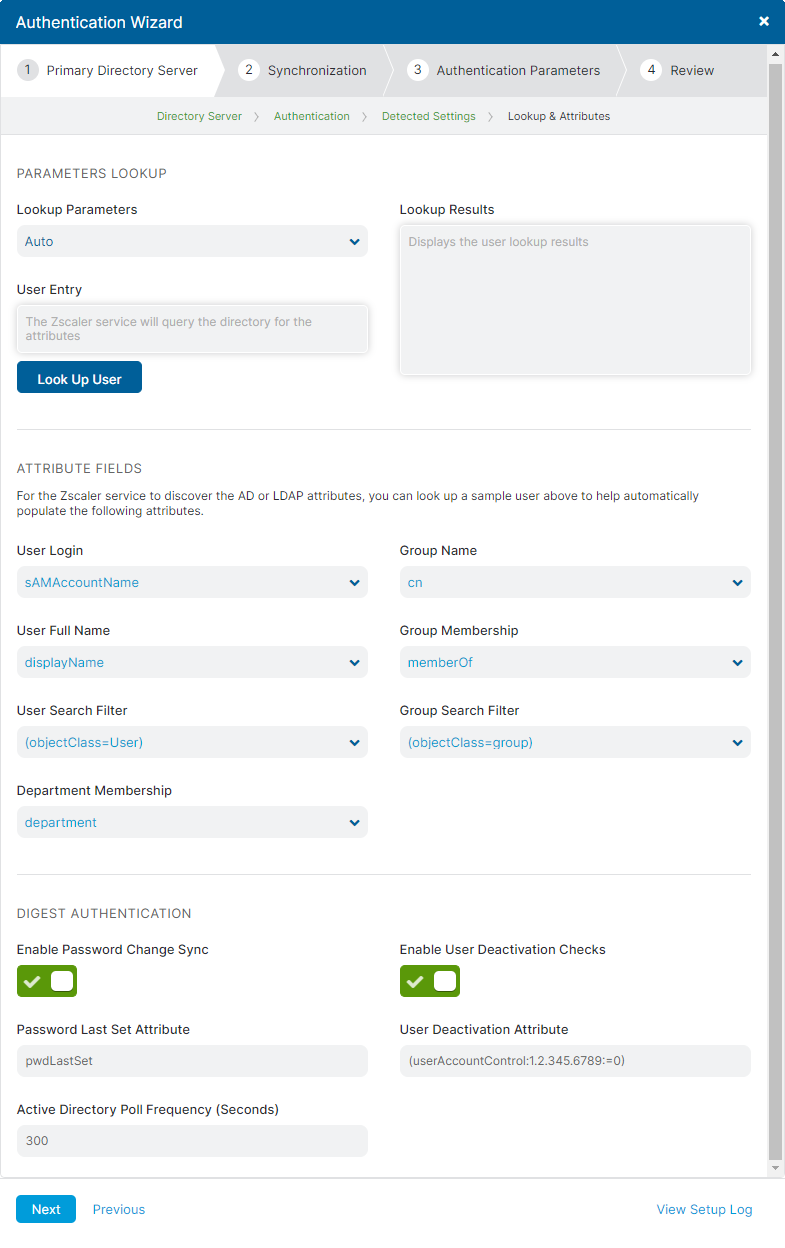The image features an interface with a structured layout for user authentication settings. The top section has a blue border with white text reading "AUTHENTICATION WIZARD," and a white "X" in the right-hand corner for closing the window. Below this border, in gray text, are sequential steps: "one, primary directory server," "two, synchronization," and "three, AUTHENTICATION parameters for review."

Highlighted in green is the text "directory server," followed by "AUTHENTICATION in detective sentence." Below this, in black, is "look up attributes." A white background with gray text reads "parameters look up," and in black, "look up parameters."

In blue text, the word "auto" is followed by "user entry" in black. An informational note states, "The Zscaler service will query the directory for attributes." Further down, a blue rectangle with white text reads "look up user." Adjacent to this, in black, is "look up results," and in gray, "display the look up results." A horizontal gray line divides these sections.

Under "attribute field" in black, there's an explanation that says, "For the Zscaler service to discover the AD or LDAP attributes, you can look up a sample user above to help automatically populate the following attributes." The fields listed are "user login" (black), "user full name," followed by "display name" in blue, and continuing in blue are "SAMA account name," "user search filter," "department membership," "group name," "group membership," and "group search filter."